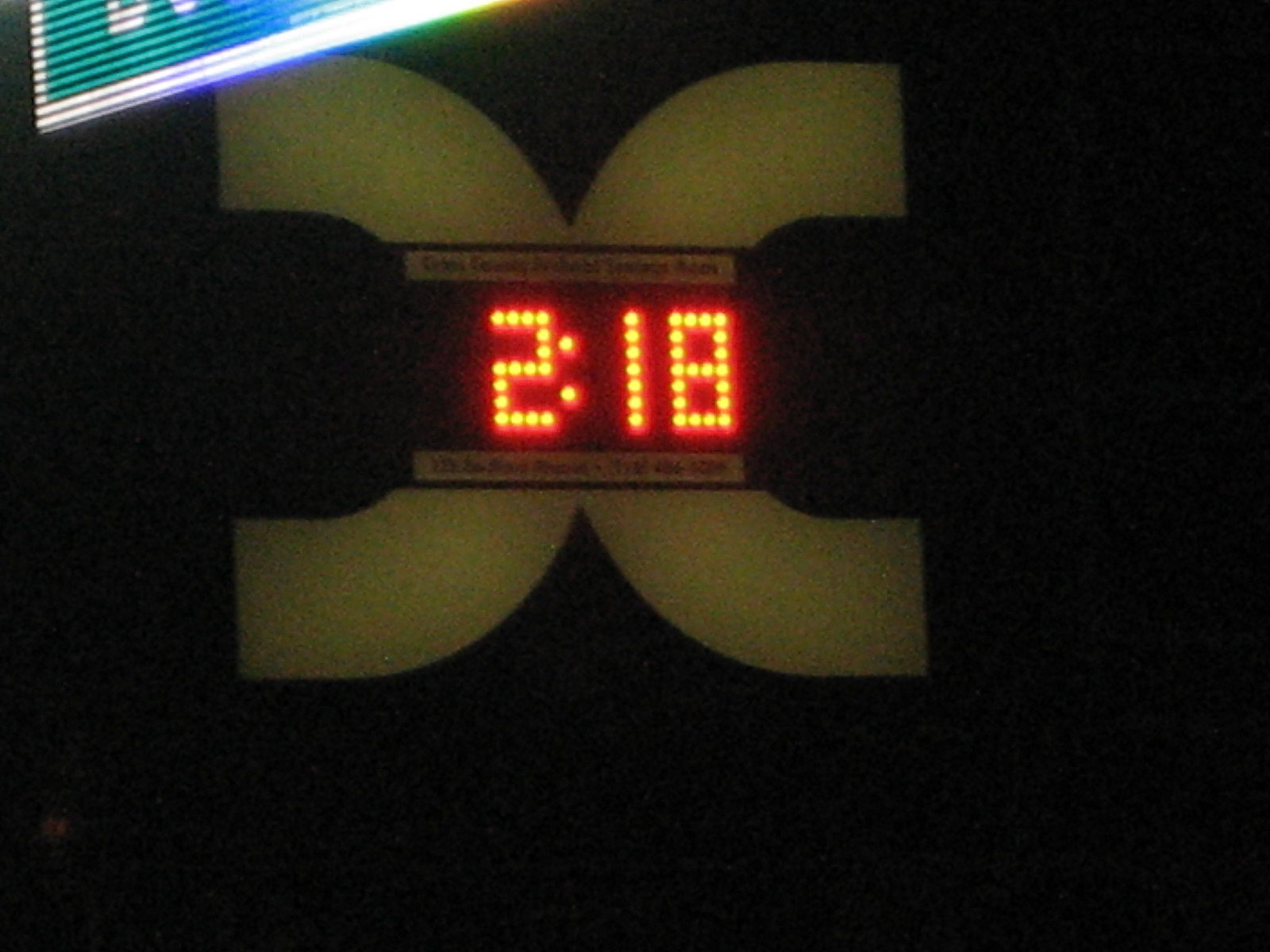The image features a predominantly black background with a prominent digital clock displaying the time "2:18" in bright, pixelated orangey-yellow numbers, reminiscent of an electronic scoreboard. Dominating the center of the image are two extremely thick tan-colored letter C's, positioned back-to-back. The left C faces left, while the right C faces right, creating a mirrored effect. Between the C's is a rectangular sign with two yellow banners—one at the top and one at the bottom—featuring dark lettering that is not clearly legible. In the top left corner of the image, there is a diagonally positioned LED sign with a white border and a turquoise-blue center, displaying white text. The sign appears slightly out of focus and exhibits the striped appearance typical of photographed digital screens. The photo captures a night-time ambiance, adding to the overall contrast and making the digital elements stand out clearly against the dark background.